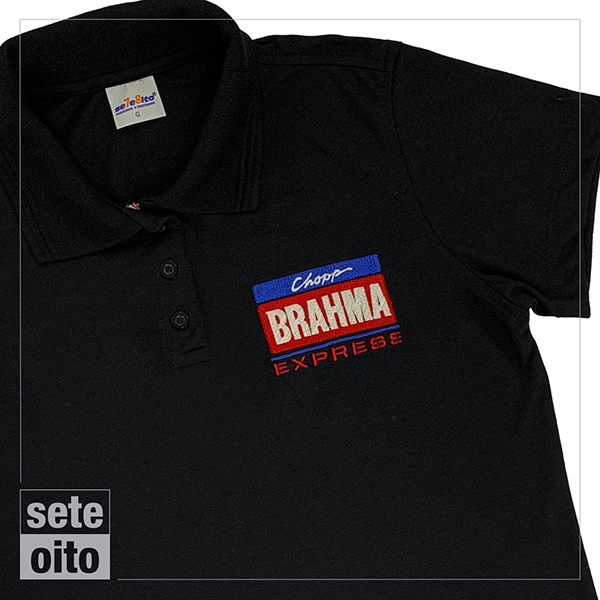This photograph captures a black polo t-shirt set against a thin gray frame that slightly overlaps the shirt's edges. The right sleeve and part of the shirt are not visible in the image. The polo features a collar and a three-button design, with all buttons fastened. The tag at the collar is white with blue and yellow text, though the specific wording is unclear. Dominating the left breast area is a prominent company logo. This logo comprises multiple elements: the text "Chart Brahma" where "Chart" is in white letters on a blue background and "Brahma" in white letters on a white background, separated by a blue stripe. Below it, "Express" is displayed in red letters without a background. A smaller box within the larger gray frame, located at the bottom left corner, shows the brand name "SETI OITO" with "SETI" in gray and "OITO" in black, indicating the likely manufacturer.